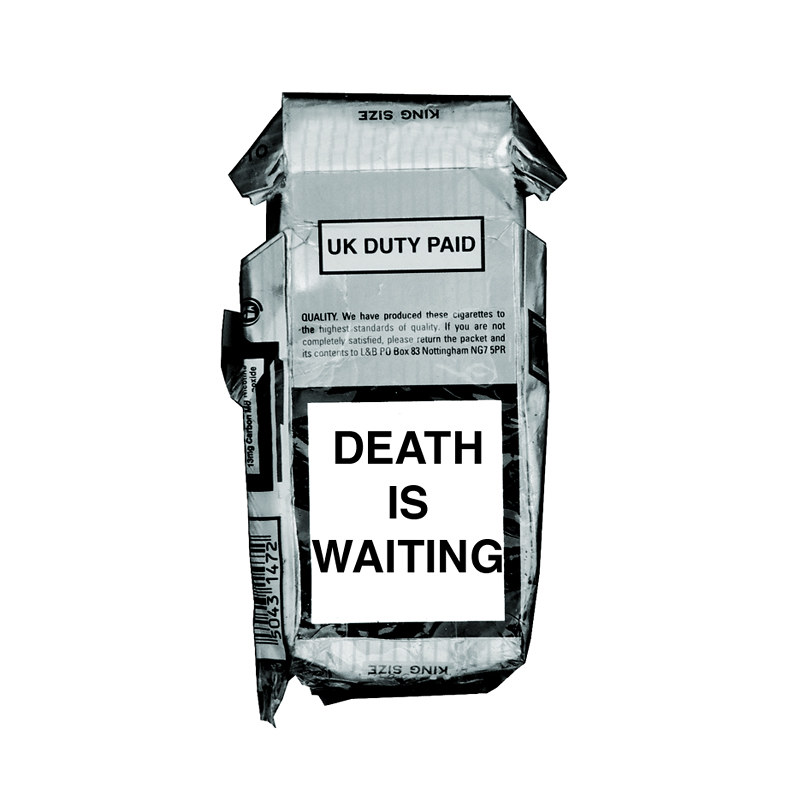This is a detailed drawing of a light blue cigarette box. The box has an irregular shape, particularly noticeable at the top and on the left side. In the middle of the box, there is text that reads: "UK Duty Paid - Quality: We have produced these cigarettes to the highest standard of quality. If you are not completely satisfied, please return the packet and its contents to L&B Peer Books, 83 Nottingham, NG7 5PR." Below this text, there is a white box with the ominous text: "Death is waiting." On the left side of the box, hints of a barcode are visible, while the right side prominently features a full barcode.